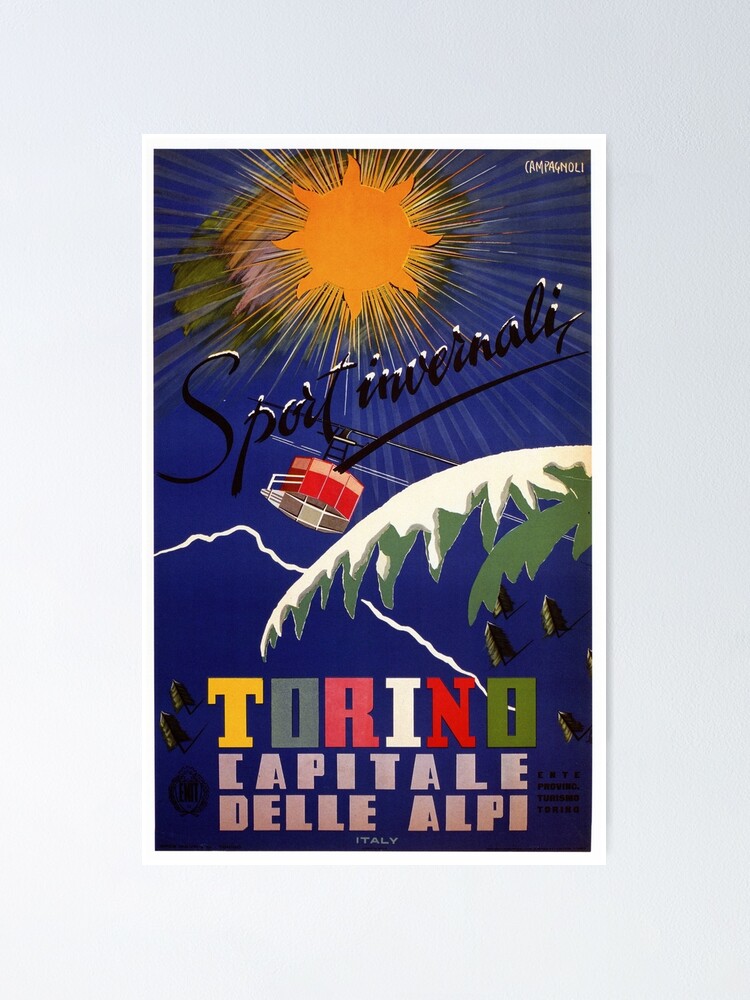This artistic print depicts a vivid poster set against a grayish textured wall with a white border around its tall blue background. Dominating the upper center of the image is a stylized, bright orange-yellow sun with rays creating a sunburst effect. Below the sun, in an elegant black cursive font with a white snow cap effect, the text reads "Sport Invernali." Encircling the upper left corner is small white text reading "Camp Ignoli."

The lower portion of the poster is vibrant and dynamic, with the phrase "Torino Capitale Delle Alpi" prominently displayed, each letter of "Torino" in a different color—gold for the T, gray for the first O, raspberry for the R, white for the I, red for the N, and olive green for the final O. The rest of the phrase is written in light pink.

Enhancing the winter feel, the image includes green palm-like leaves with snow components, stylized white lines depicting snow-covered mountains, angled tree graphics, and a red ski lift or gondola moving across the scene. The entire composition artfully combines these elements to evoke a lively winter sports ambiance in Italy's alpine capital, Torino.